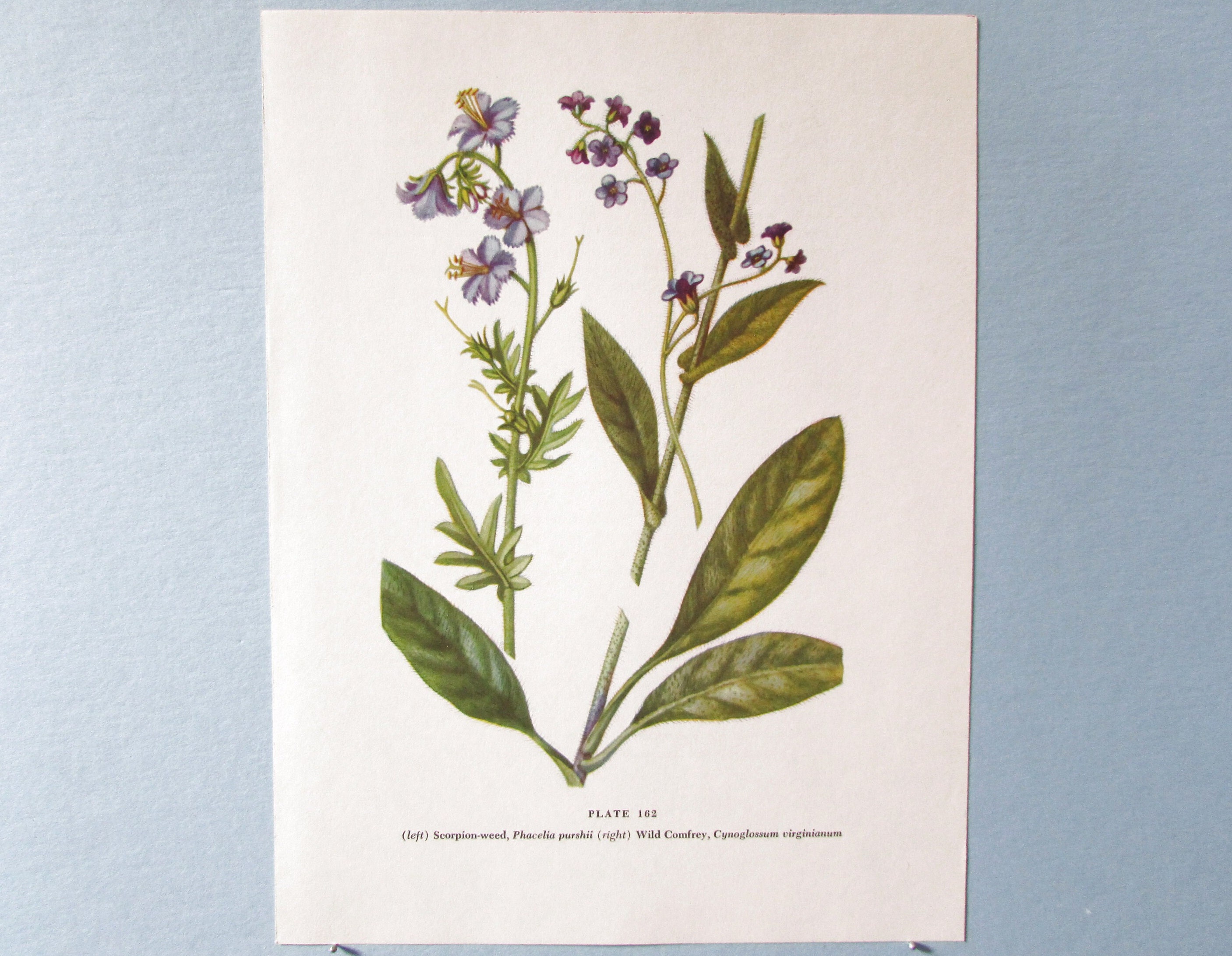This rectangular image features a realistic, yet intricately drawn colored pencil illustration of two flowering plants on a white background. The artwork is attached to a light blue-gray wall, gradually lightening towards the left as if subtly illuminated. The drawing is secured by two small silver pins at the top corners. 

At the bottom of the image, there's clear black text that reads: "Plate 162. Left: Scorpion Weed (Phacelia percyi). Right: Wild Comfrey (Cynoglossum virginianum)." The depiction showcases the plants in detail: vibrant green leaves and stems support clusters of light violet and dark purple flowers. The flowers, though realistically rendered, might appear smaller and more delicate than their real-life counterparts, giving the impression of a botanical illustration or field study.